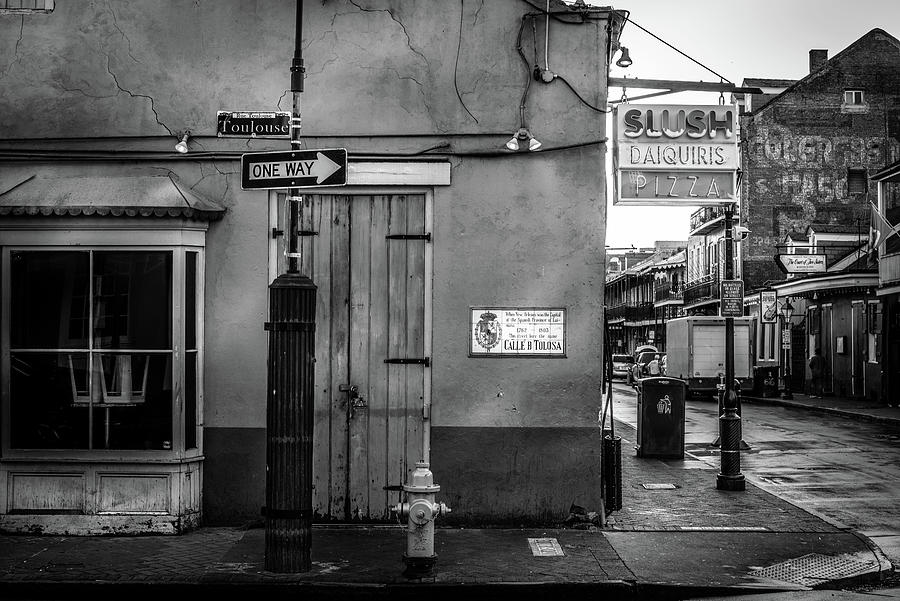This is an old black and white photograph of a narrow city street, possibly in France, given the prominent street sign labeled "Toulouse". The main focus is a one-story stucco building with a wooden door adorned with metal latches and a bay window revealing darkness inside. A one-way sign points to the right in front of this structure. There is a white sign with a dark frame on this building, which appears to read "Calais Toulouse," although its exact wording is unclear. A hanging sign on the building advertises slush, daiquiris, and pizza, suggesting it might be a restaurant. The street is littered with a trash can and a large truck parked, contributing to a slightly dirty appearance. To the right, the street continues with various vehicles parked alongside, lined with predominantly two-story brick buildings featuring railings. The photo captures a slice of city life from a bygone era, showcasing distinctive architectural elements and street furniture like a fire hydrant and an array of informative signs.